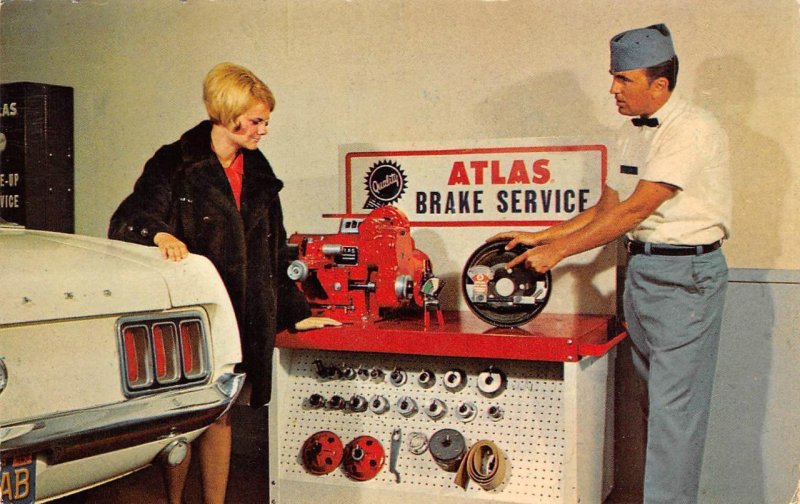In this vibrant color photograph, likely from the 1950s or 60s and possibly an advertisement, a man and woman are positioned on either side of a red-topped work table, engaging with automotive parts in what appears to be a demonstration for Atlas Brake Service. The woman, standing on the left, is adorned in a thick fur coat with a blonde bob hairstyle, and she rests her hand on the trunk of a white car, which is visibly elevated as if being worked on. She is also dressed in what seems to be a red blouse or dress and has bare legs. Opposite her, the man, who sports a white short-sleeve button-up shirt with a black bow tie, blue dress pants, a black belt, and a blue hat reminiscent of a soda jerk's cap, points at or demonstrates a wheel or gear atop the table. Behind them, a sign on the wall reads "Atlas" in red and "Brake Service" in blue, with additional tools neatly organized on a pegboard beneath a cabinet. The scene underscores an instructional interaction, indicative of mid-century automotive culture.